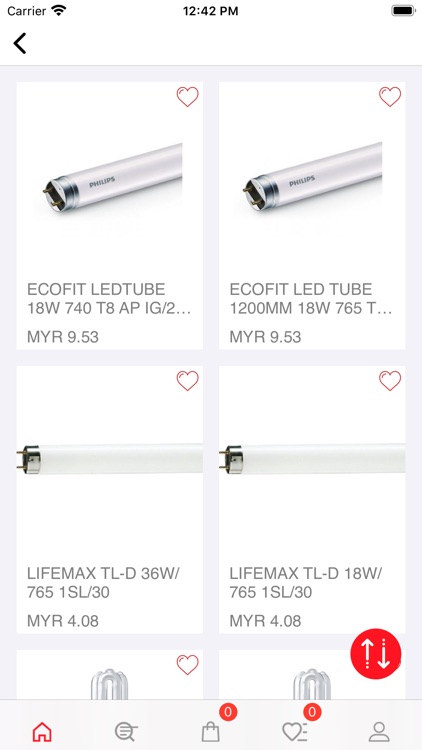The image is a screenshot of a sales application interface. At the top of the screen, in the upper left corner, there is a label showing "Carrier" next to three full Wi-Fi signal bars. The current time, displayed in the center, reads 12:42 p.m. On the upper right corner, a fully charged battery icon is visible. 

The first item listed is "Ecofit Lead Tube 18W 740 T8 AP IG," with part of the description cut off, priced at MYR 9.53. Next is a similar item, "Ecofit Lead Tube 1200mm 18W 765," also partially cut off. 

Following these, two items labeled "Lifemax TLD" are shown. On the left side, there's "36W 765 1SL30," and on the right side, "18W 765 1SL30." Both are priced at MYR 4.08.